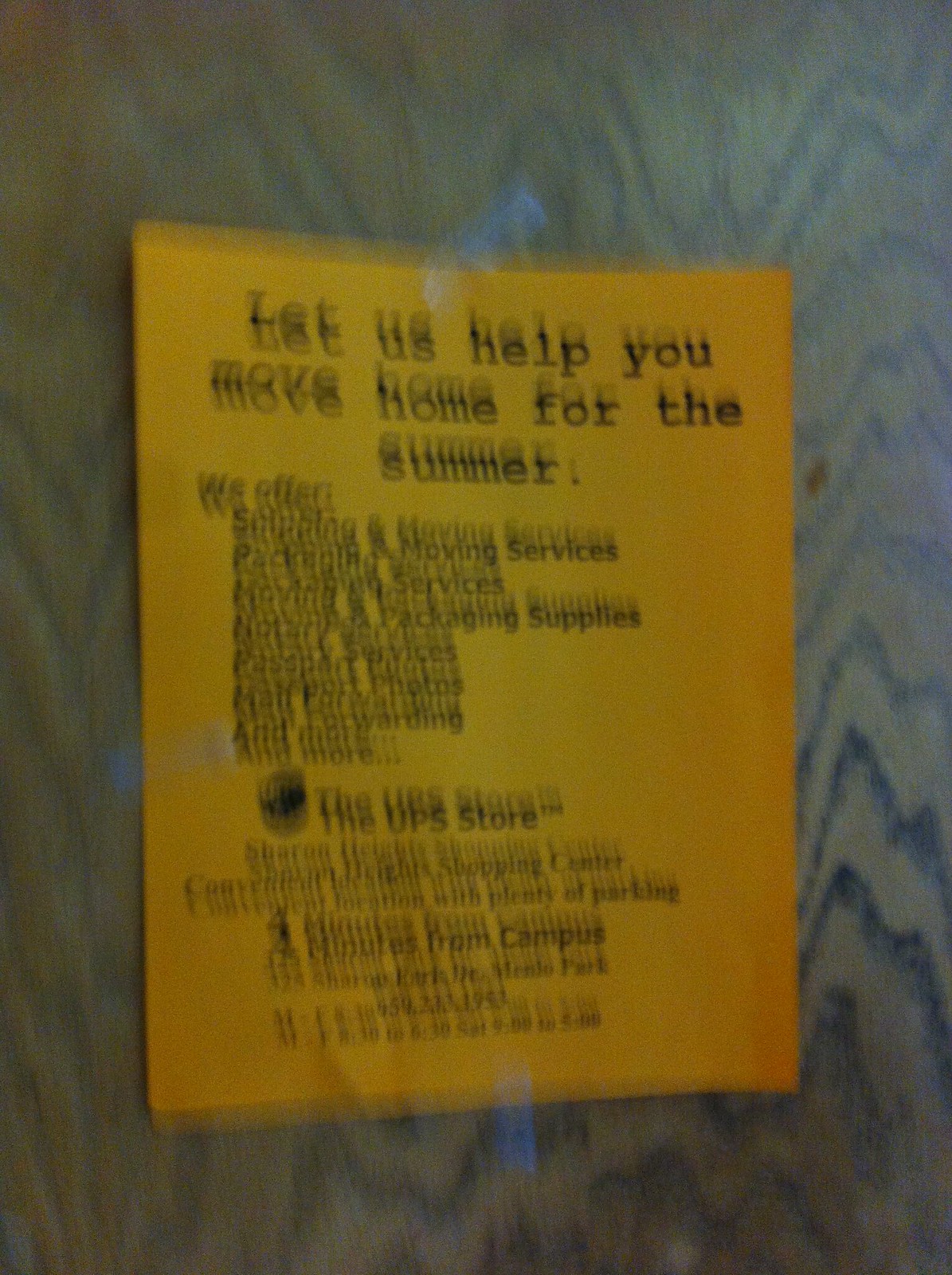The image depicts a somewhat blurry yellow flyer taped to a wall with clear tape on the bottom, left, and upper sides. The wall features a light blue swirl pattern. The flyer, printed with black text, is titled, "Let Us Help You Move Home for the Summer." It offers services such as shipping and moving services, packaging services, moving and packing supplies, notary services, and passport services. The flyer prominently features the UPS Store logo and states it is located at the Sharon Heights Shopping Center, just four minutes from campus, indicating its convenience for university students. The flyer also provides additional location details, possibly mentioning Menlo Park, New Jersey, or universities like NJIT or Princeton.